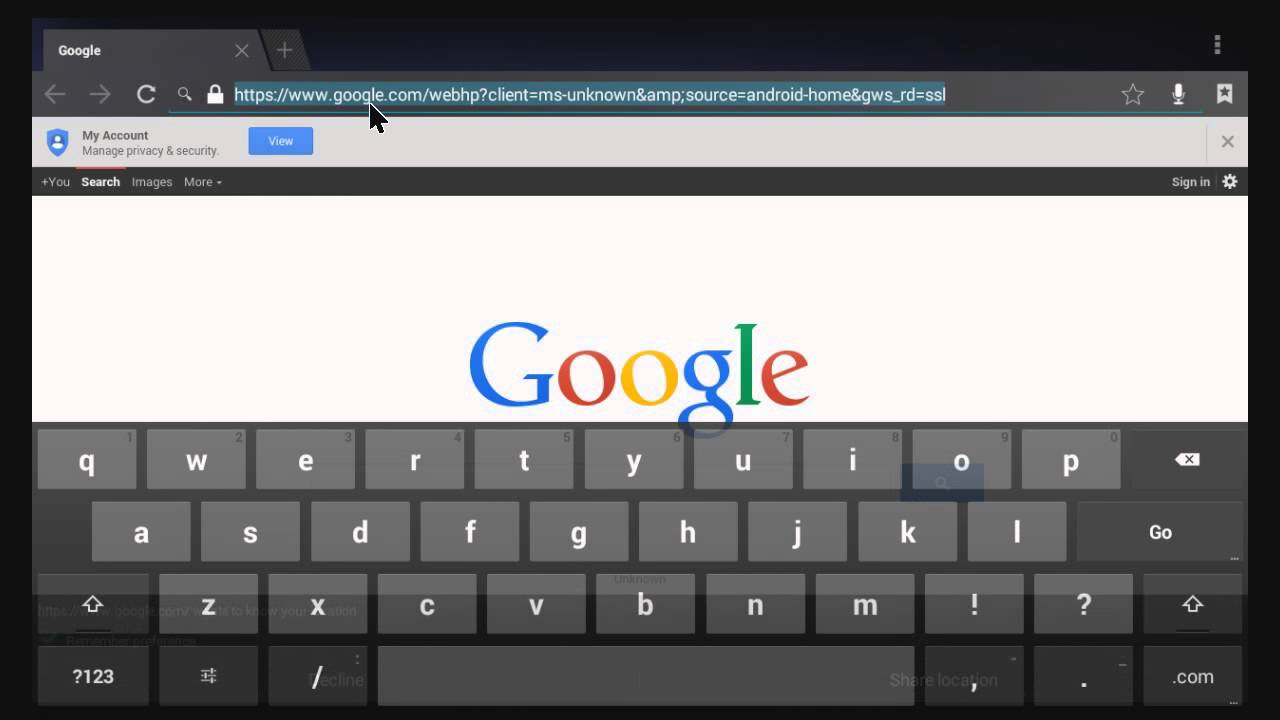This is an image capture of a computer screen displaying the Google homepage. At the top of the screen, the URL bar shows the web address: `https://www.google.com/webhp?client=ms-unknown&source=android-home&gws_rd=ssl`. Below the URL, there are several options visible including "My Account" and "Manage Privacy and Security," accompanied by a blue shield icon with a person symbol inside it. Next to these, there is a blue-clickable box labeled "View."

Prominently displayed in the center of the screen is the iconic Google logo with its multicolored letters: a blue capital "G," followed by a red lowercase "o," a yellow lowercase "o," a blue lowercase "g," a green lowercase "l," and a red lowercase "e."

At the bottom portion of the screen, there is a virtual keyboard layout, similar to what one would see on a physical computer keyboard, but displayed on the screen itself, likely indicating touch-based input.